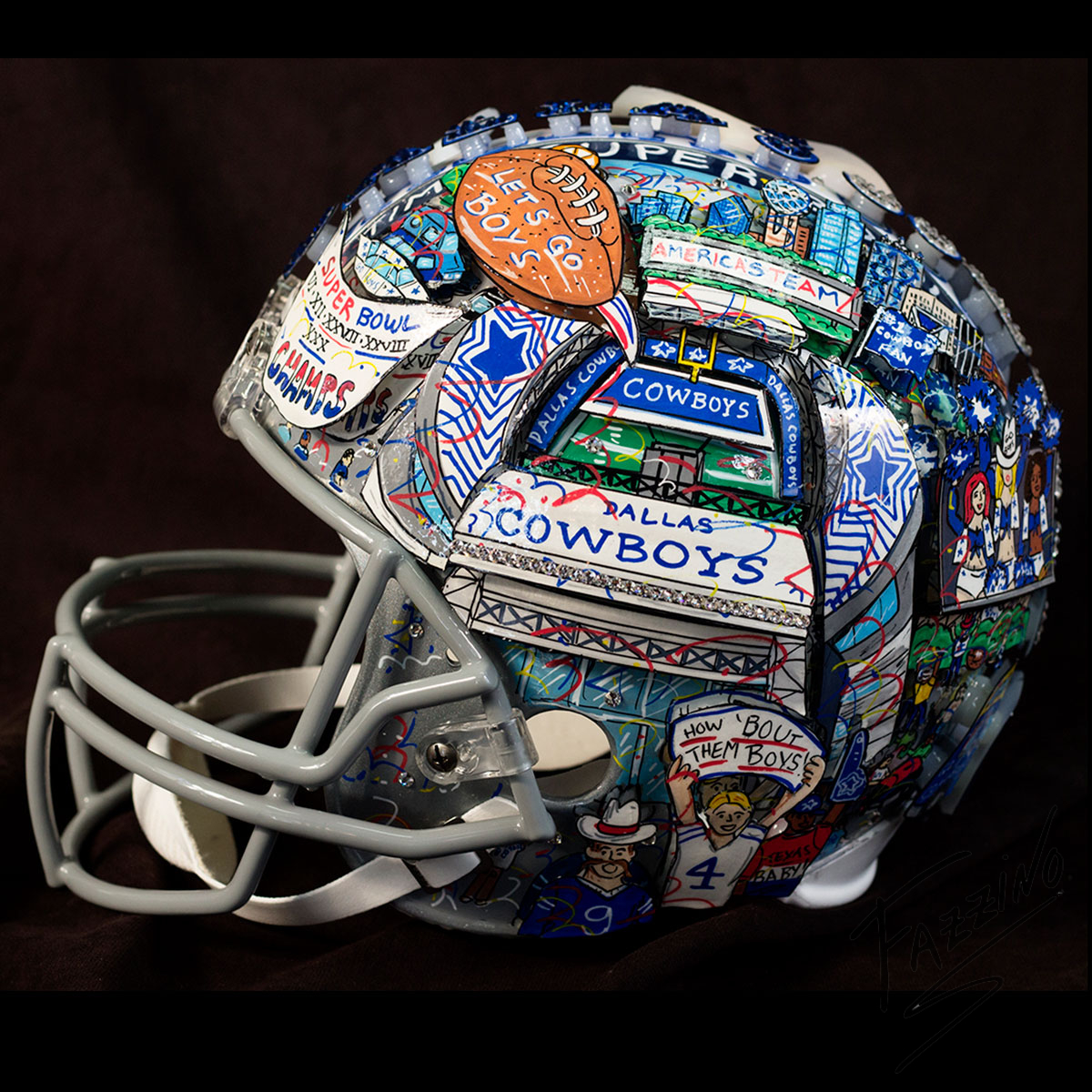This color photograph, in a square format, showcases a decorated Dallas Cowboys football helmet prominently positioned at the center of the image. The helmet is a vibrant collage of various designs and images, rich in detail and color. Predominantly, the helmet features hues of blue, gray, brown, and white. The left profile of the helmet is vividly visible, displaying an array of caricatures, symbols, and text.

At the front of the helmet, a gray face mask covers the mouth and nose, complemented by a white chin strap. Directly above, set against a white background, the words "Dallas Cowboys" are written in bold blue letters. Further up, a silhouette of a football field with a gold goal post stretches towards the top of the helmet, with the word "Cowboys" written in white on a blue background in this area.

A prominent brown football illustration with the phrase "Let's Go Boys" in white text is positioned toward the top of the helmet, showcasing detailed stitching. Just below this football, another banner reads "Super Bowl Champs" with Roman numerals in red and white letters. 

Drawings of cheerleaders in blue and white outfits, revealing midriffs, adorn the back of the helmet. Additionally, a caricature of a fan holds up a banner with the phrase "How About Them Boys." The bottom section of the helmet, under the ear area, displays the number four holding the aforementioned banner. Another drawing shows a cowboy-headed figure in a blue jersey with the number nine.

The helmet also features rows of raised buttons along the hairline, running down the center ridge. The background of the photograph is black, emphasizing the multicolored and intricate patterns on the helmet and capturing the essence of photographic representational realism.